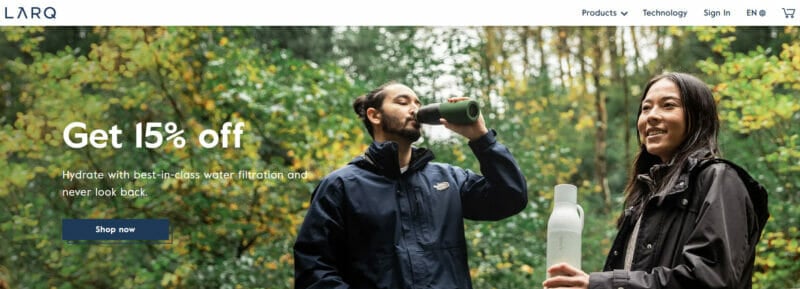The image features a detailed advertisement for LARQ at the top left corner in capital letters. On the top right, there is a horizontal navigation menu with the options: 'Products,' 'Technology,' 'Sign-In,' 'EN,' and a shopping cart icon.

The main advertisement image depicts an outdoor scene under a slightly overcast sky, filled with a diverse forest landscape composed of trees of varying heights and colors, ranging from dark green to light green, and some with yellow-tinged foliage. 

In the foreground, white text reads "Get 15% off" and promotes the product with the phrase "Hydrate with best-in-class water filtration and never look back." Below this, a blue banner invites viewers to "Shop Now."

The scene includes a man and a woman situated to the right. The man, dressed in a navy blue windbreaker, is shown drinking from a thermos. The woman, attired in a black jacket, holds a clear water bottle in her hand, adding to the emphasis on hydration solutions showcased in the ad.